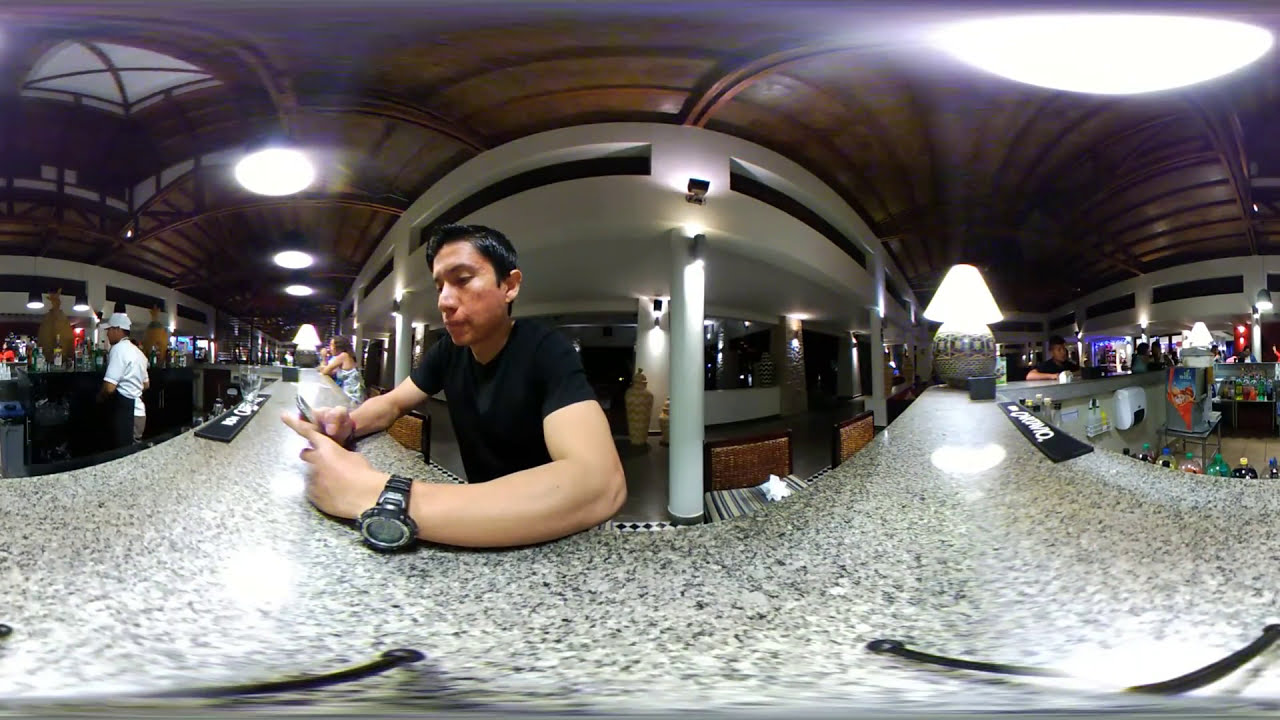The photograph captures a Hispanic man with short black hair, dressed in a black t-shirt and wearing a prominent black watch on his left wrist, as he sits at a speckled granite countertop in what appears to be a well-lit restaurant or bar. The man is intently focused on his cell phone. The countertop, a mix of grey, white, and black speckles, extends throughout the scene, creating a cohesive backdrop. To his right, the bar area features various drink bottles, including sodas and likely alcoholic beverages, arrayed under hanging ceiling lamps that brighten the entire bar area. Beyond him, patrons continue down the elongated bar, with some seats occupied and others empty. White pillars descend from the ceiling soffit, adding structural interest to the setting. A man in service attire—a white shirt and a white hat—stands to the right, possibly preparing food or drinks. Further in the background, a woman with brown hair, dressed in white, is seated at the counter, adding to the lively yet orderly atmosphere of the restaurant.